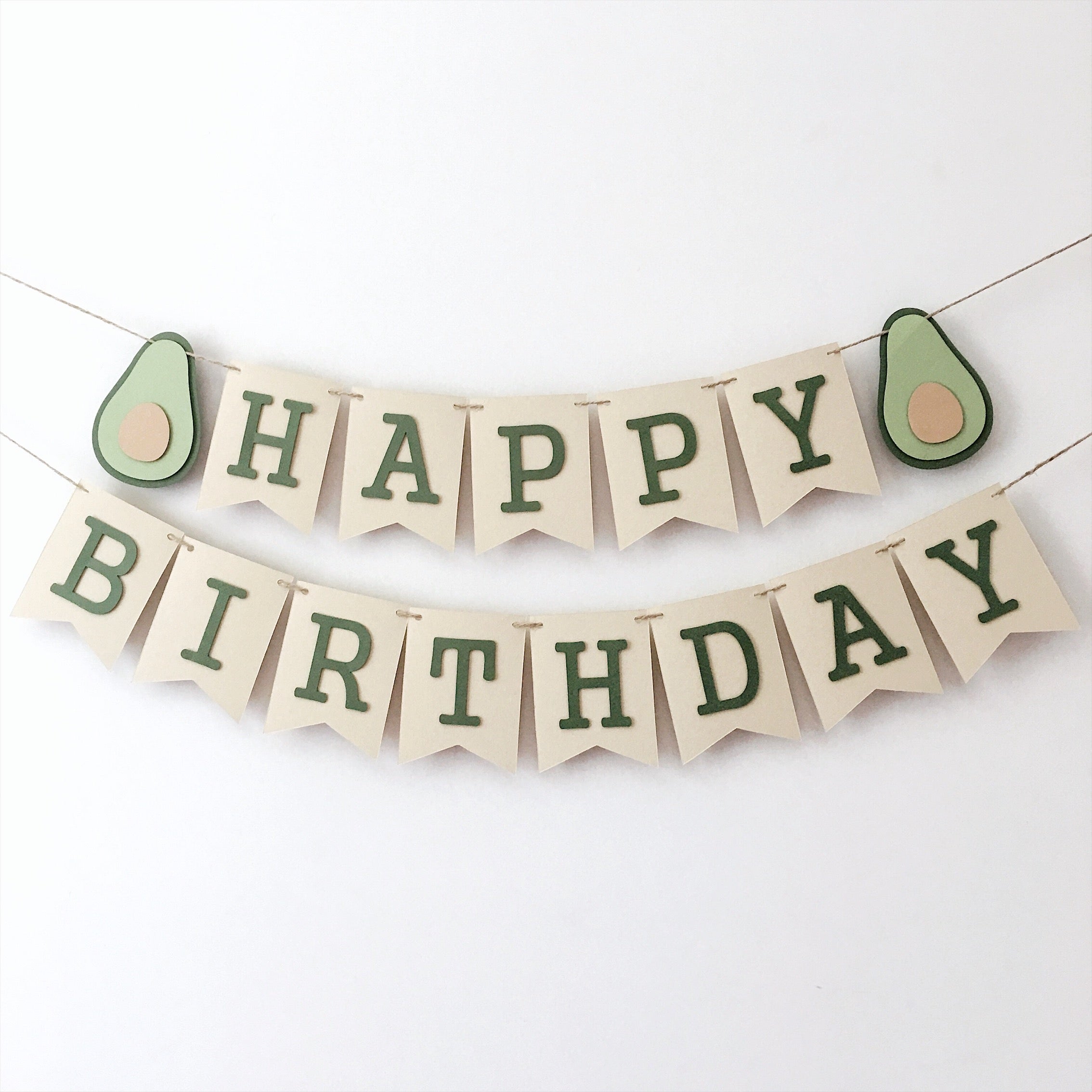The image showcases a creative art project designed to say "Happy Birthday." Displayed against a light background that transitions from white on the left to light gray in the center and darker gray on the right, the project consists of two hanging strings adorned with decorative elements. The top string features a series of beige cards with green letters spelling out "HAPPY," flanked by two styrofoam avocado shapes—one beside the "H" and one beside the "Y." Beneath this, the bottom string holds similar beige cards which spell out "BIRTHDAY" in green lettering. Each avocado is painted green with a brown center, and the avocados, as well as the letter cards, may potentially be magnets. Designed in a charming and visually appealing manner, this "Happy Birthday" banner is ideal for hanging up in a home environment, such as on a wall or refrigerator, to celebrate someone's special day.